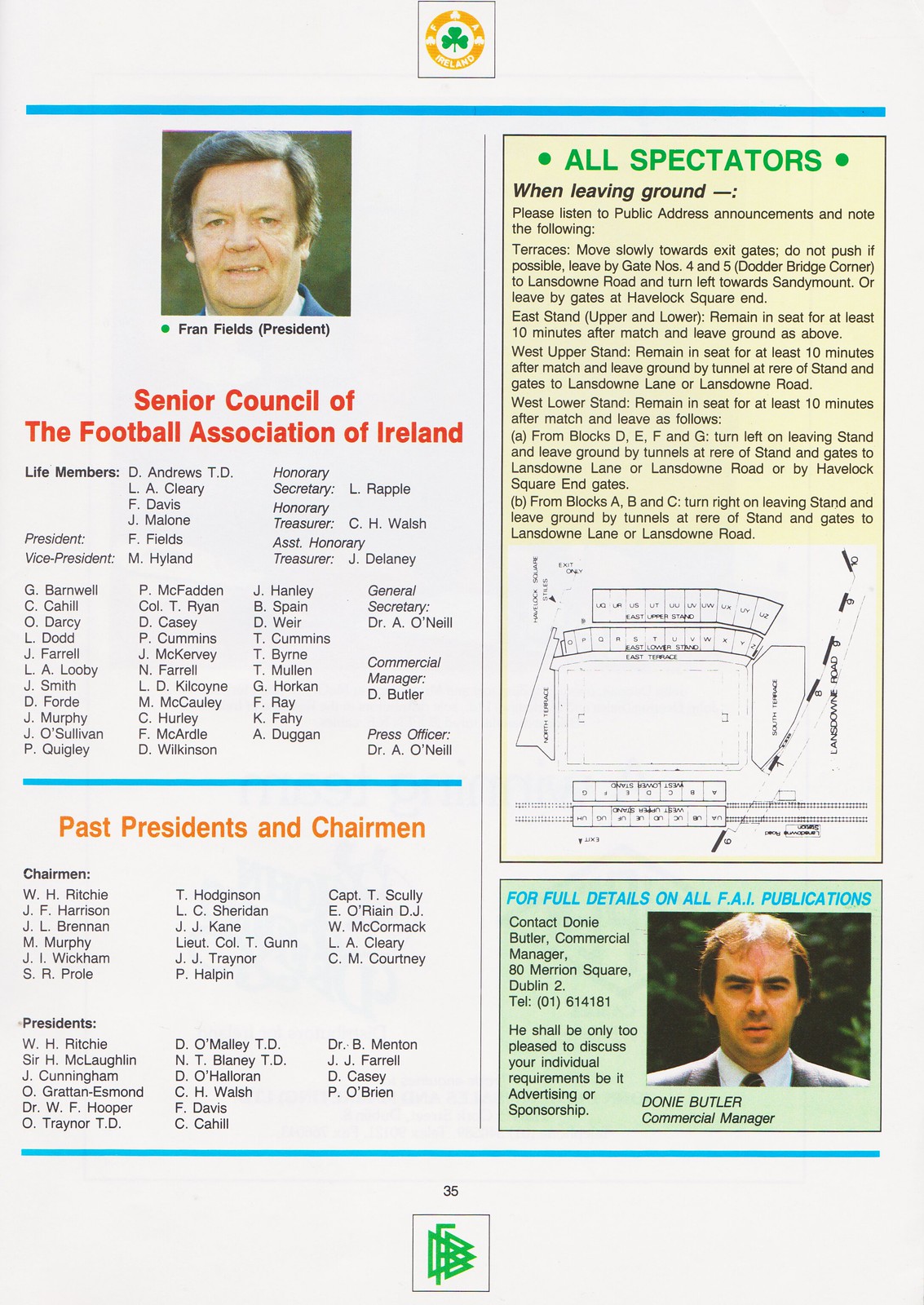This vertically aligned rectangular image appears to be a page from a magazine or an appendix, predominantly with a white background. At the top center, there is a gold circle with a cloverleaf—the logo. Below the logo, a headshot of a man with a smirk is displayed, identified as Fran Fields (President). Beneath his photo, red text reads "Senior Counsel of the Football Association of Ireland," followed by a list of life members in black font. 

A blue line separates this segment from the next section, which is titled "Past Presidents and Chairmen" in orange text. This section contains lists of names under the subheadings "Chairmen" and "Presidents," both in black font.

On the right side of the image, there is a green title saying "All Spectators." Below it, directions for spectators when leaving the ground are provided in black text. This includes instructions to listen to public address announcements, move slowly towards the exits, and specific directions for the East and West stands. Under these instructions, there is a black-and-white outline of a stadium, likely a seating chart.

Finally, at the bottom right corner, a section titled "For full details on all FAI Publications" in blue text is presented. Here, a photo of a man named Donnie Butler, identified as the Commercial Manager, is included, along with contact information.